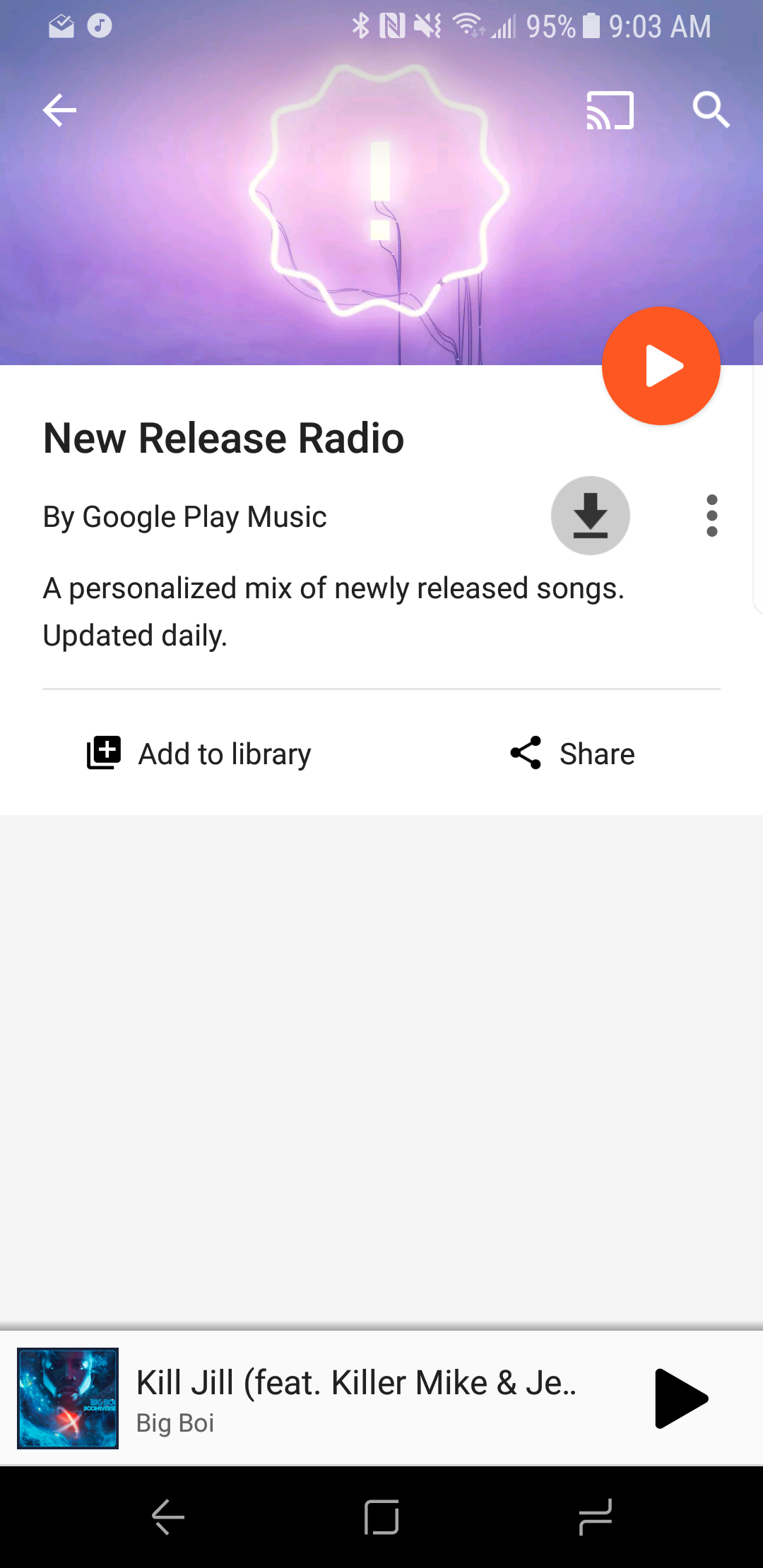The screenshot captures a mobile device's interface with multiple notification and status icons at the top. 

**Top Section:**
- An enclosing row at the top displays various icons: 
  - An envelope icon.
  - A small white circle containing a music note.
  - Bluetooth, Near Field Communication (NFC) (depicted as a white box with an "N"), a speaker icon with a slash through it (indicating mute).
  - The Wi-Fi symbol and signal strength.
  - The battery level at 95% and the time displayed as 9:03 AM.

**Central Section:**
- The central area features a lavender background with a prominent white starburst graphic in the middle, encapsulating a white exclamation mark.
- On one side, there are additional icons: a white square with lines, symbolizing content/document, and a magnifying glass icon, representing search.
- On the other side of the lavender background, there is a white arrow and an orange circle with a white play button.

**Main Content:**
- Below the lavender background, the main section presents a white background with black text describing "New Release Radio by Google Play Music", which is a personalized mix of newly released songs updated daily.
- Adjacent to the "by Google Play Music" text is a gray circle with a black arrow, beneath which lie three vertical gray dots.
- Further down, red text reads "Add to Library" accompanied by two square icons with a plus sign. It says "Share" next to a small arrow symbol.

**Bottom Section:**
- The bottommost part showcases a thin white box containing the black text of a song title: "Kill Jill featuring Killer Mike and J.E...," where the rest of the title is cut off. The artist is identified as Big Boi (spelled as B-I-G-B-O-I).
- Alongside the song title, there is a black arrow.
- Below this information, a black thin strip is visible with icons: a white arrow, a white square, and two white owl-like figures.

The screenshot merges functionality with an appealing UI, portraying music recommendations and actions such as adding to the library or sharing, clearly showcasing how users interact with music content on Google Play Music.